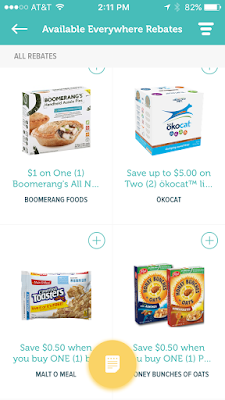This image is a screenshot from a coupon application, showcasing various rebate offers. At the top of the screen, there's a greenish-blue banner displaying essential phone details. The time is 2:11 PM, indicated in white numbers. The phone's battery level stands at 82%, the location services are enabled (as shown by the location arrow), and the device is connected to AT&T with three bars of signal strength. The Wi-Fi connection is active, denoted by the Wi-Fi icon.

Below the banner, a message reads, "Available Everywhere Rebates." Underneath this message, four distinct rebate offers are presented:

1. **Boomerang All-Natural Meal** - $1 off one item. The accompanying image shows a Boomerang meal box featuring a pot pie on the cover.

2. **Ökocat Cat Litter** - Save $5 on the purchase of two boxes. The image displays a box with the Ökocat logo and a picture of a cat.

3. **Malt-O-Meal Cinnamon Toasters Cereal** - $0.50 off. The visual representation includes a box of the cereal.

4. **Honey Bunches of Oats Cereal** - Save $5 on the purchase of one box. The image shows a box of Honey Bunches of Oats cereal.

This detailed screenshot provides a clear and comprehensive look at the available rebate offers and essential phone details.